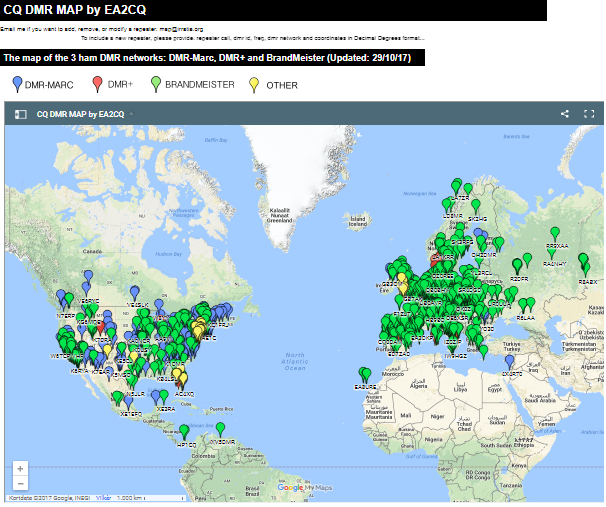This screenshot captures the CQ DMR map by EA2CQ, prominently displayed at the top in a black bar. Below this title, there is a body of text rendered in black font. Another black bar follows, stating, "Map of the three ham DMR networks: DMR-MARC, DMR Plus, and BrandMeister (updated 29-10-17)."

The map itself is a detailed world map, showcasing North America, Europe, Africa, South America, the Middle East, Iceland, the Atlantic Ocean, and parts of the Pacific Ocean on the left side. The legend for the map is included, where different colored pins represent the various DMR networks: a blue pin for DMR-MARC, a red pin for DMR Plus, a green pin for BrandMeister, and a yellow pin for "Other."

In North America, the map is dotted with numerous green, blue, and some yellow pins highlighting the presence of multiple networks. Europe is primarily marked with green pins, with a few blue pins interspersed. Central America features a small scattering of pins, and there are individual pins in both North and South America, near Africa, and a single blue pin in the Middle East.